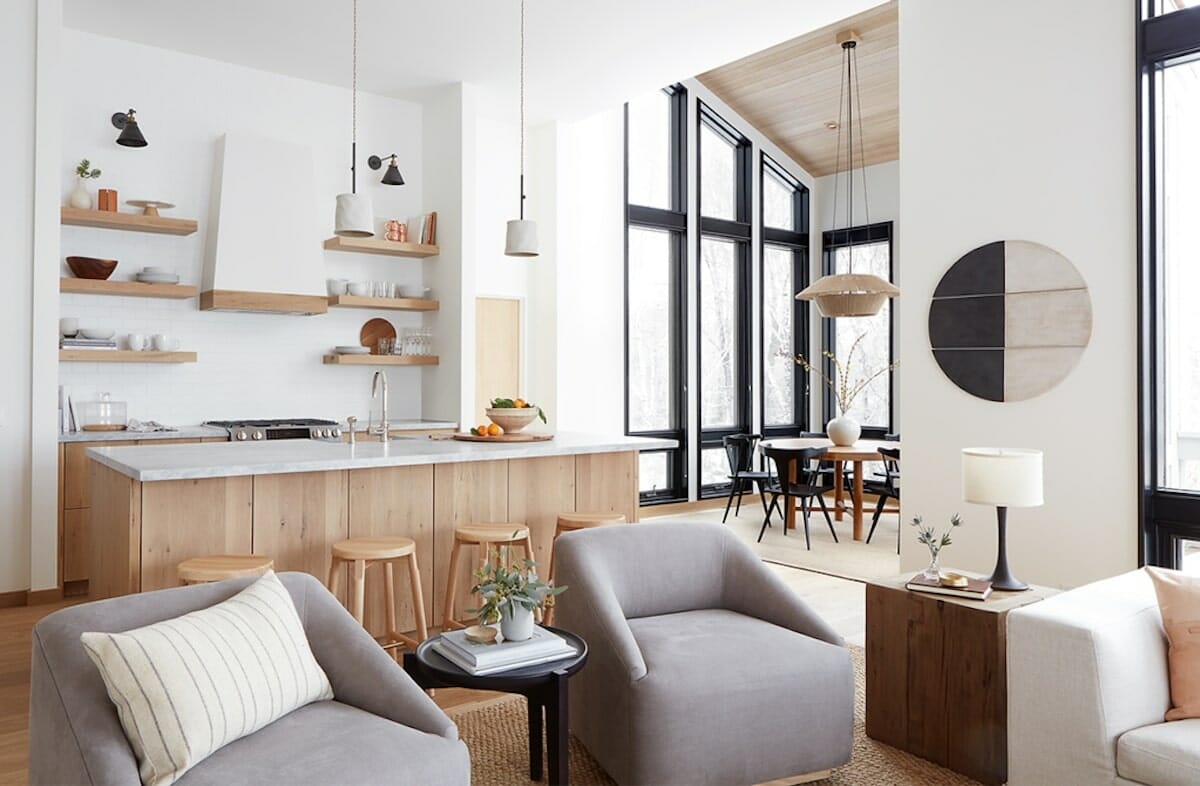This image depicts a stylish and modern living room that seamlessly transitions into a dining and kitchen area. The room features pristine white walls and a rich hardwood floor, partly covered by a tan carpet. In the foreground, two gray armchairs are positioned with an off-white pillow on the left chair and separated by a small black round end table, which holds a book and a white potted plant. On the right, there's a glimpse of a white sofa accompanied by a dark brown cube table with a lamp atop it.

The background reveals an open kitchen area distinguished by light wood cabinets and shelves, with a white marble countertop. The kitchen island, topped with a white surface and surrounded by four light pine stools, is illuminated by two pendant lights with white lampshades hanging from the ceiling. A chrome-colored gas range with black burners and a hood is partially visible, and six light wood shelves on the back wall display various dinnerware.

To the left, the image captures an alcove functioning as a dining area with tall, floor-to-ceiling windows showing a wintry outdoor scene of snow-covered trees. This area houses a brown circular table surrounded by a couple of black metal chairs and features a striking tan chandelier hanging from the slanted ceiling. The table also has a white vase with decorative plumes as a centerpiece. The overall setup exudes a refined, magazine-like elegance.